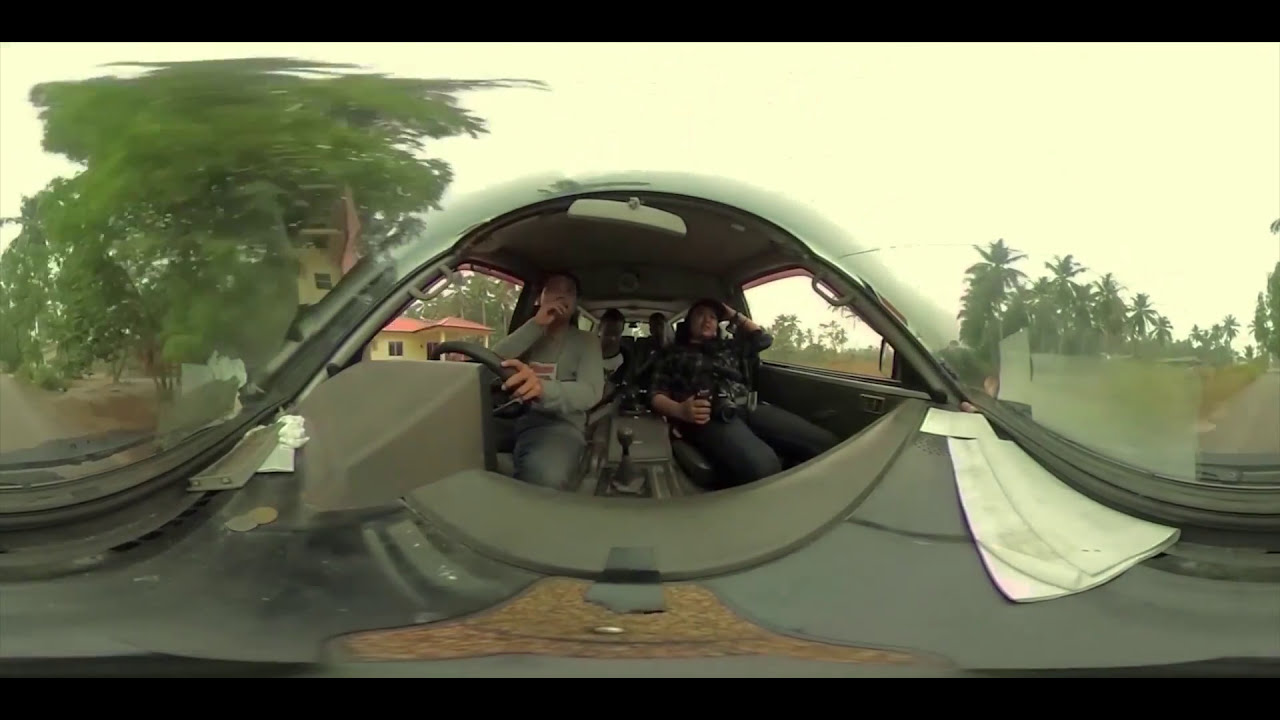This detailed color photograph uses a fisheye lens and a panoramic filter to create a composite image of a military vehicle with a rounded, khaki green exterior. Inside the vehicle, which is viewed straight into the cockpit, there are four men in uniform. The driver, wearing a gray, long-sleeved shirt, has his hand on the steering wheel on the left side. Next to him, in the passenger seat, is a man in a darker uniform holding a camera. Behind them, two more men are partially visible. The vehicle's windshield, framed by a rearview mirror and dashboard, faces outward towards a scenic background. To the left, there is a large green tree in front of a stucco house with a red tile roof. On the right, a paved road lined with tropical-looking trees and grass extends into the distance. The sky is overcast, adding a white hue that contrasts with the green landscape and the vehicle's color. The photo's horizontal orientation and the black strips across the top and bottom enhance its panoramic, representational style.